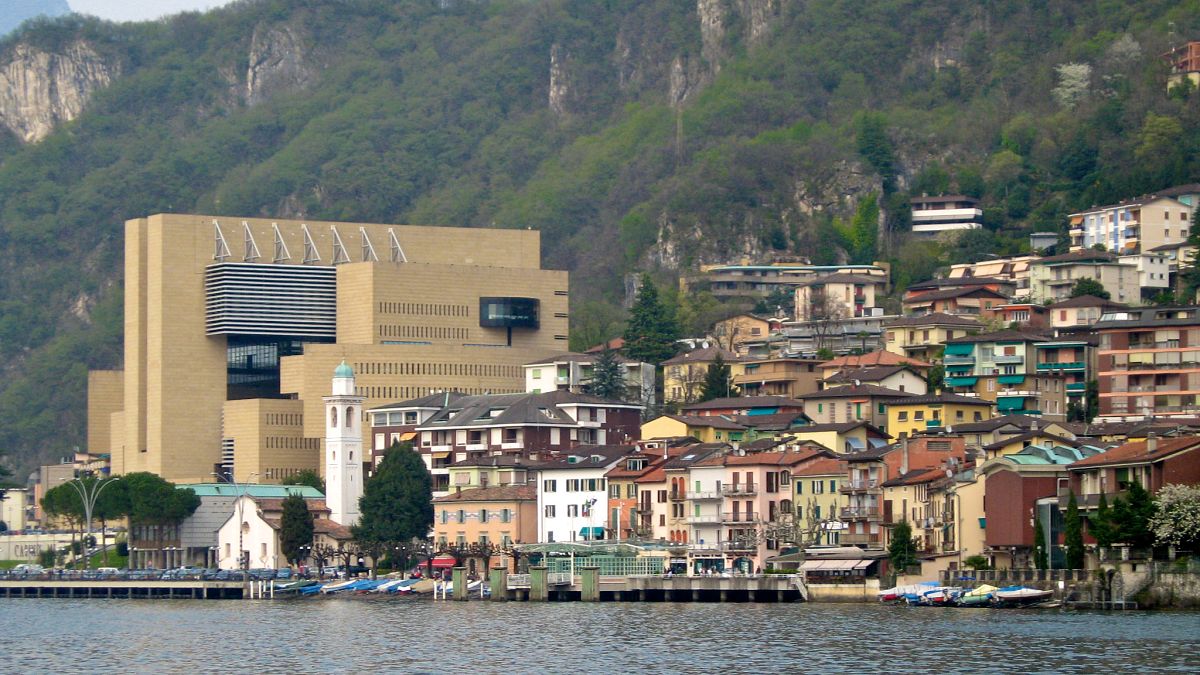The photograph showcases a picturesque cityscape featuring a sea-facing property set against a lush natural backdrop. The multi-storied buildings, which include modern apartment complexes and hotels, are primarily brown and stand in stark contrast to traditional European-style houses with sloping roofs. The structures are arranged in a triangular pattern on an inclined hillside. Dominating the left part of the image is a prominent yellow rectangular building with uniquely assembled rectangular sections. Adjacent to this, a church and a tower, possibly a lighthouse, are visible, with cars parked in front of the church. The densely forested mountains with luscious green trees form a scenic backdrop. The greenish, glistening water body at the bottom of the image reflects the city's vibrancy. Numerous boats can be seen, particularly in the center and to the right of the image, enhancing the harmonious blend of urban and natural elements.